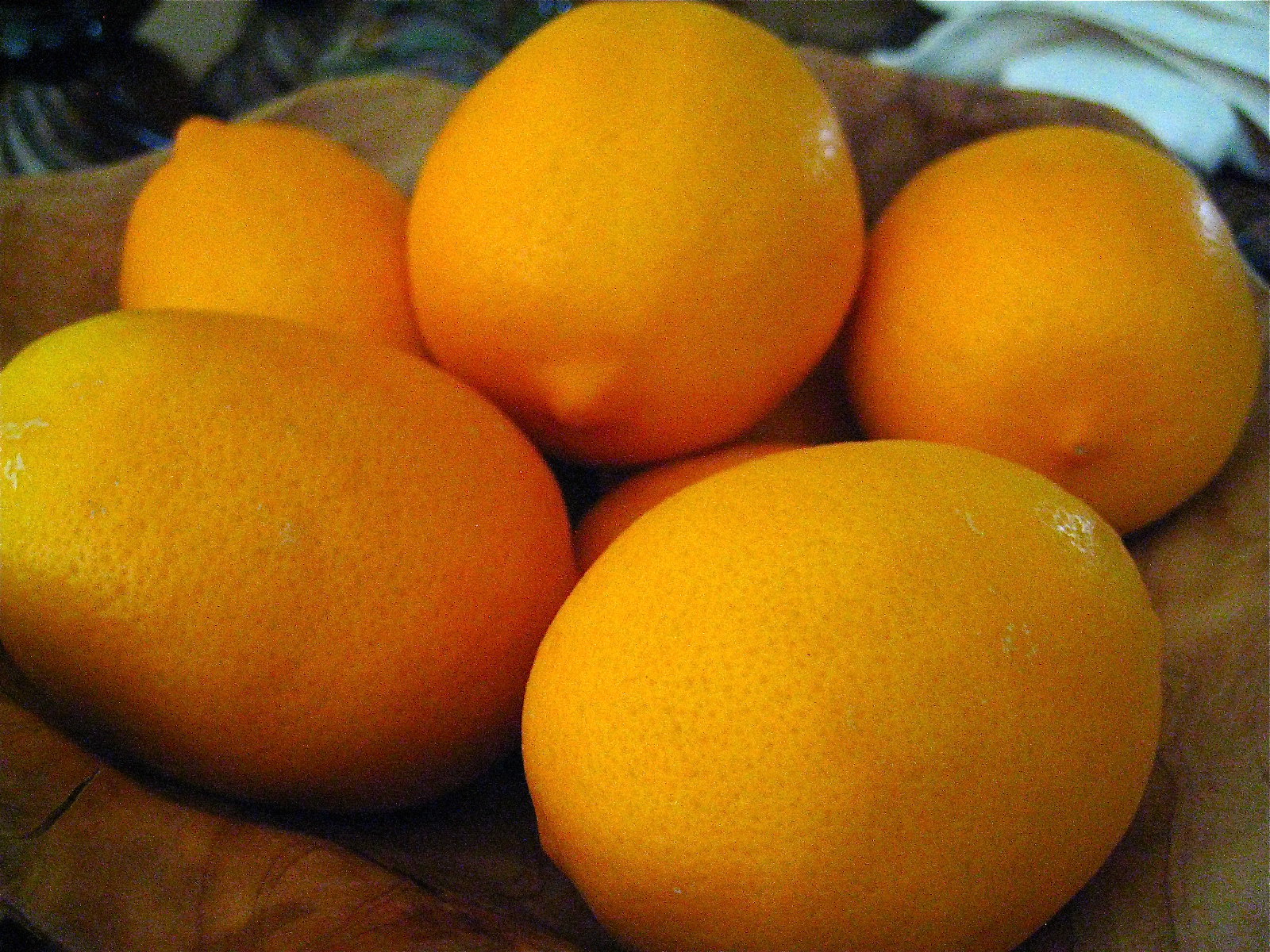This close-up image captures around six large, ripe lemons arranged in a rustic, medium-colored wooden bowl. The wooden bowl, which appears well-maintained and possibly stained, cradles the lemons in a somewhat circular formation, with one lemon prominently perched atop the others. The lemons are a vibrant, almost orange-tinted yellow, marked with small black circles and indents on their skin, and each lemon features a characteristic nub or bump at its end. The scene is set in a dimly lit room, as indicated by the blurred background and the soft white light reflecting off the lemons' glossy surfaces. Overall, the image has a grainy quality, likely due to being captured with a lower-quality camera.